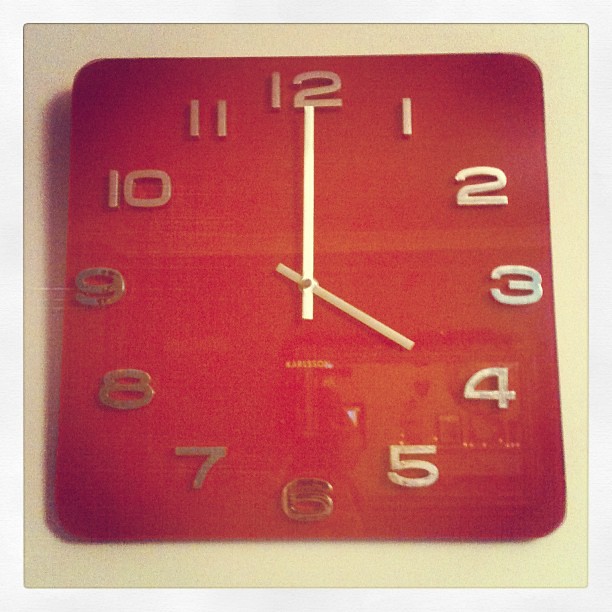The image features a square, red clock mounted against a light-colored wall, which appears to be either white or tan. The clock displays silver-colored numerals from 1 to 12 and has hands that are a silvery-white hue, indicating the time as 4 o'clock. The wall around the clock is darker, casting distinct shadows on the left side. The background of the photo has dark corners shading to black. A reflection on the clock face reveals a scene with a small shelf on the opposite wall, adorned with three picture frames.